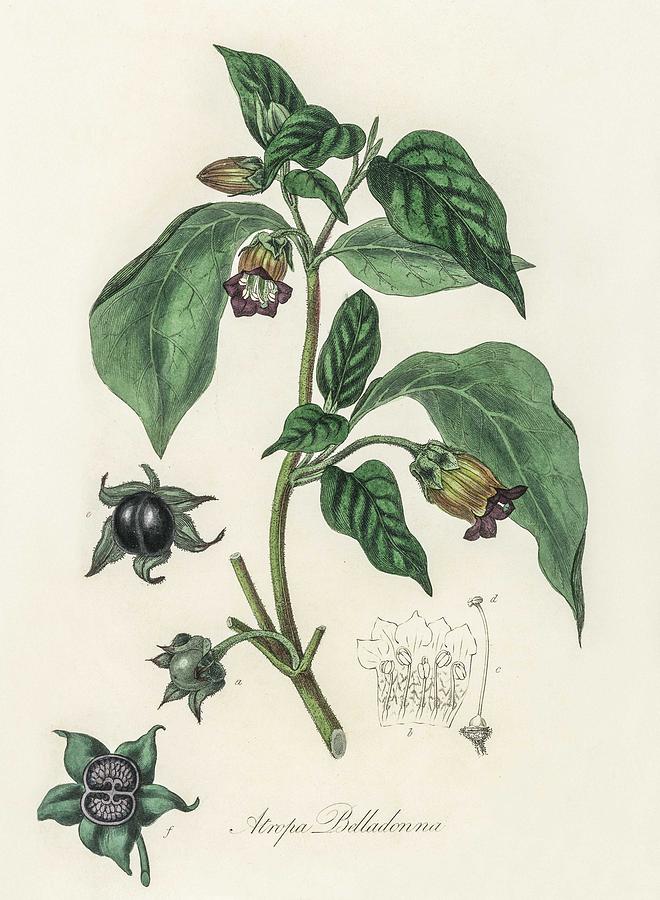This is a detailed botanical illustration of the plant Atropa belladonna, indicated by a cursive inscription at the bottom of the page. The background is a cream color. The main element is a stem of belladonna, adorned with several sets of leaves, which are an amalgam of dark green and lighter green stripes on top, and plain green beneath. The illustration displays two open flowers; one about a third of the way up the stem, facing to the right, and another two-thirds up, facing to the left. The flowers exhibit a yellow or brown exterior and transition to a purple and white, or brown, interior. Additionally, there is an unopened flower near the top. On the left side of the page, there are two images of seed pods: one is an intact black sphere with a central line, positioned above a cut-open version revealing numerous small white seeds inside. Below the main flower and slightly above the text, there is a rough sketch of a cross-section of a belladonna flower, further contributing to the detailed depiction of the plant.